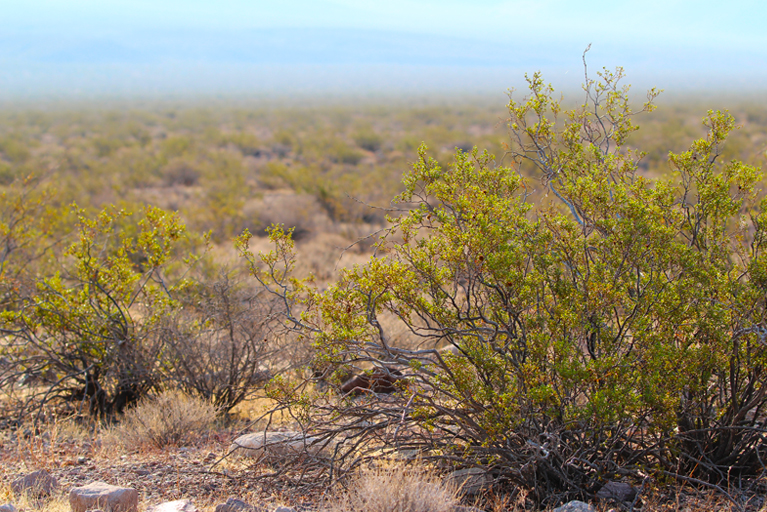The image captures a desolate, arid landscape characterized by a combination of brown and green short plants covering most of the ground. In the foreground, there are several short green bushes with very thin branches, alongside a scattering of stones in light brown and dark brown hues. Gray rocks also punctuate the barren terrain. The scene exudes a sense of dryness and desolation, with sparse tumbleweed-like bushes and dried grasses dominating the view. As the eye moves towards the horizon, the ocean becomes visible, although it appears hazy and indistinct. Beyond the ocean lies a faint, barely discernible mountain range, merging with the blue but blurry sky. The overall impression is one of a parched, thirsty landscape extending endlessly towards a distant, indistinct horizon.